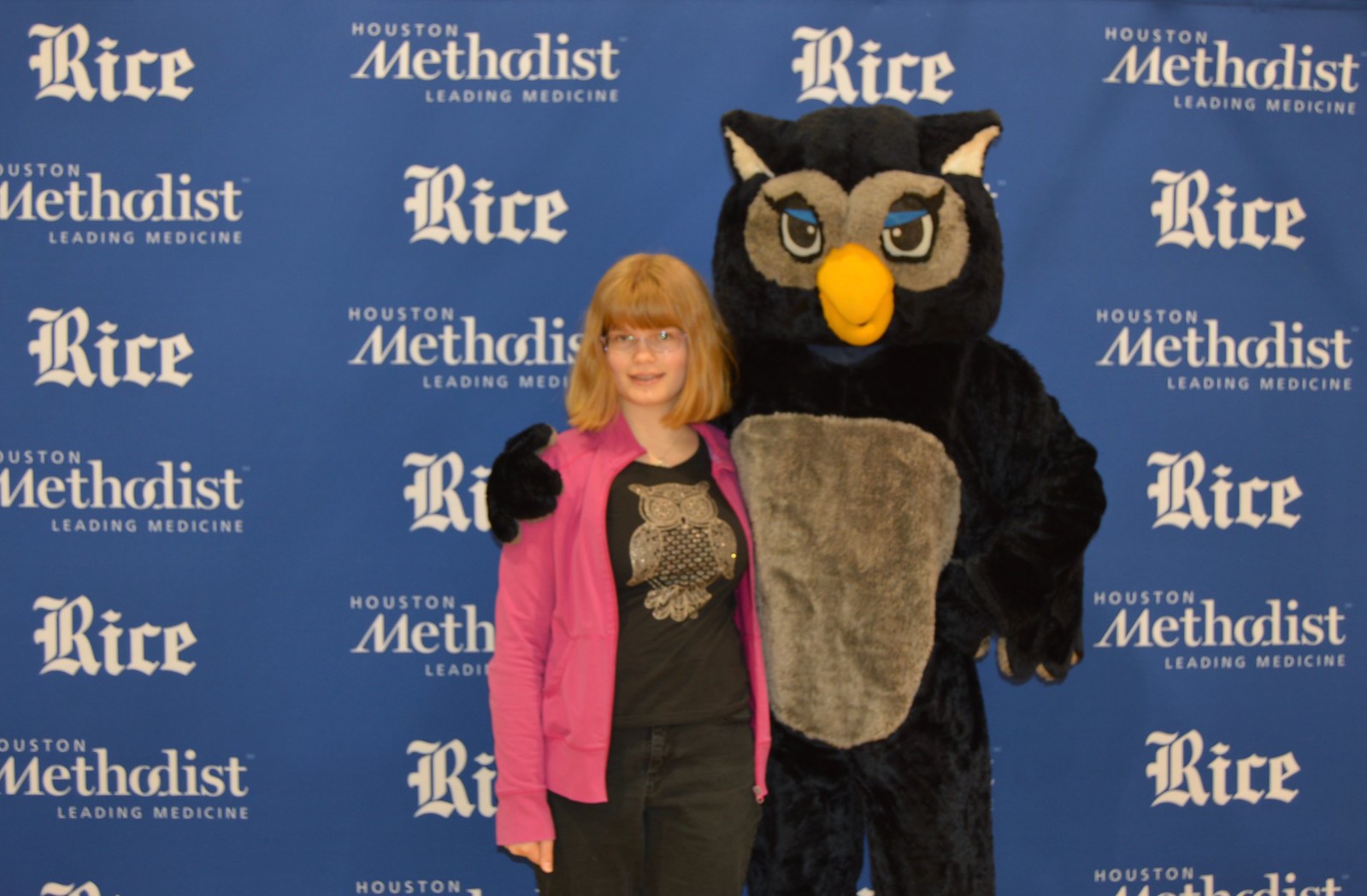In this vibrant image, a middle school-aged girl with shoulder-length red hair, bangs, and glasses is seen posing at Rice University beside their owl mascot. They stand against a striking blue backdrop filled with repeated logos: one bearing "Rice" in a gothic-style font, and the other stating "Houston Methodist Leading Medicine" in white text. The young girl, dressed in a black t-shirt featuring an owl design, a red zip-up sweater worn open, and black jeans, smiles warmly at the camera. The mascot, a black owl with a tan belly, tan accents around its eyes and ears, blue eyelids, and a yellow beak, stands cheerfully beside her, creating a perfect keepsake of her day at the university.